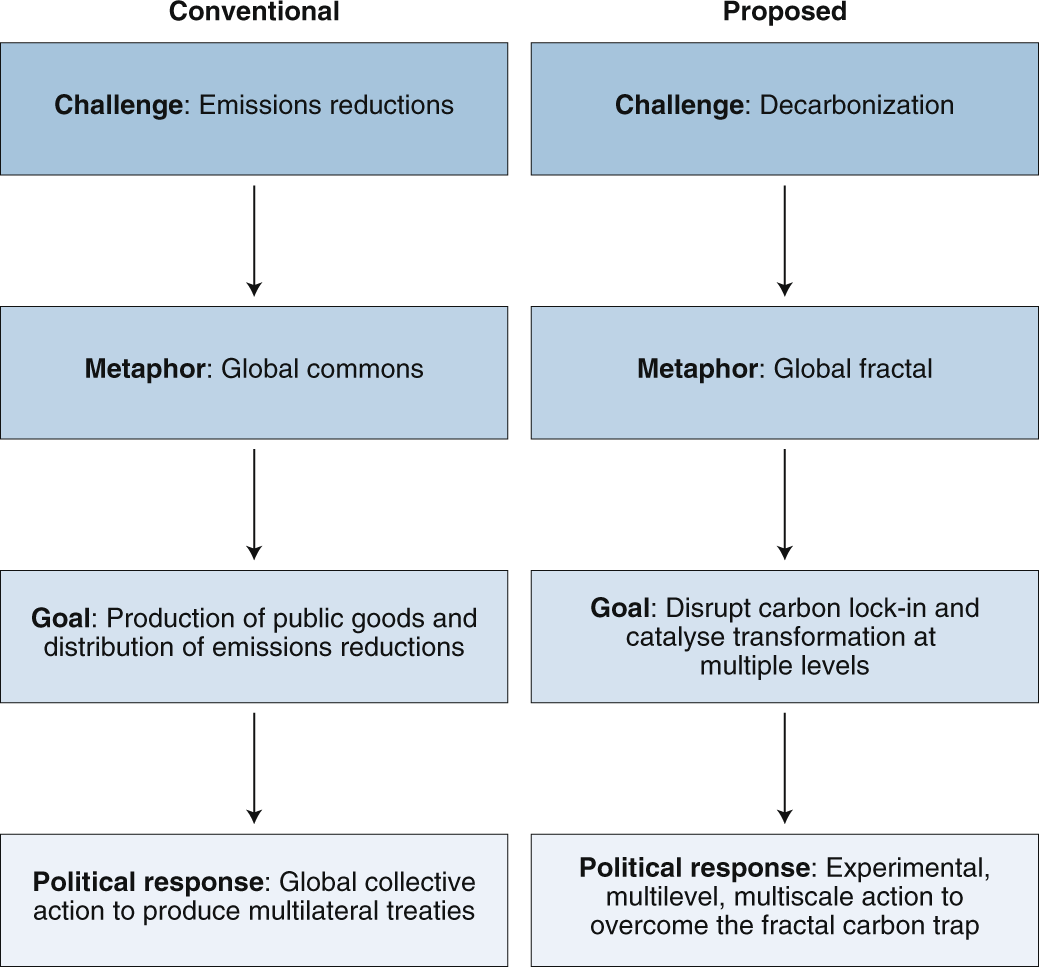This image features a detailed side-by-side comparison of two vertically-aligned flow charts against a white background. Each flow chart consists of four rectangular boxes, with an ombre effect transitioning from darker blue at the top to almost white at the bottom, connected by black arrows pointing downward. 

The left flow chart is titled "Conventional" in bold black letters. The four boxes, from top to bottom, contain the following text: 
1. "Challenge: Emissions Reduction"
2. "Metaphor: Global Commons"
3. "Goal: Production of Public Goods and Distribution of Emission Reduction"
4. "Political Response: Global Collective Action to Produce Multilateral Treaties"

The right flow chart is titled "Proposed" in bold black letters. The four boxes, from top to bottom, contain the following text:
1. "Challenge: Decarbonization"
2. "Metaphor: Global Fractal"
3. "Goal: Disrupt Carbon Lock-in and Catalyze Transformation at Multiple Levels"
4. "Political Response: Experimental, Multilevel, Multiscale Action to Overcome the Fractal Carbon Trap"

The design emphasizes a comparative perspective between traditional and innovative approaches to addressing environmental challenges, with a clear progression of ideas articulated within each chart.